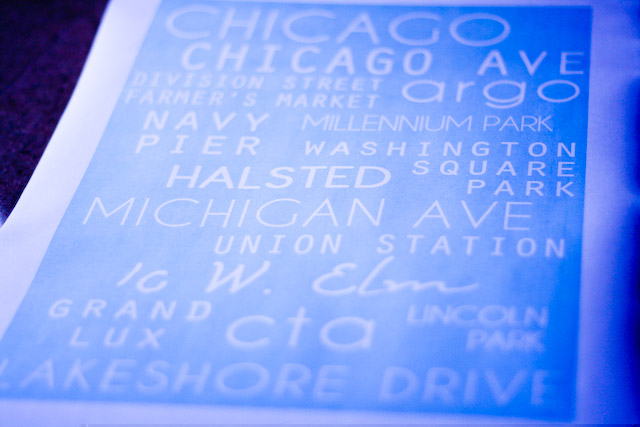This image depicts a sign featuring a vibrant blue background with a gradient effect, transitioning from darker to lighter blue, against which a piece of white-bordered paper is positioned at an angled perspective, creating an upward tilt in the photograph. The sign is adorned with an eclectic mix of place names associated with Chicago, each rendered in varying fonts, sizes, and arrangements, adding to the chaotic yet charming appearance. Prominent locations listed include Chicago, Chicago Ave, Division Street, Farmers Market, ARGO, Navy Pier, Millennium Park, Washington Square Park, Halstead, Michigan Ave, Union Station, and 10 West Elm in cursive script, among others. Additional places mentioned are Grand Lux CTA, Lincoln Park, and Lakeshore Drive. The layout suggests an artistic representation of Chicago's diverse and iconic destinations.